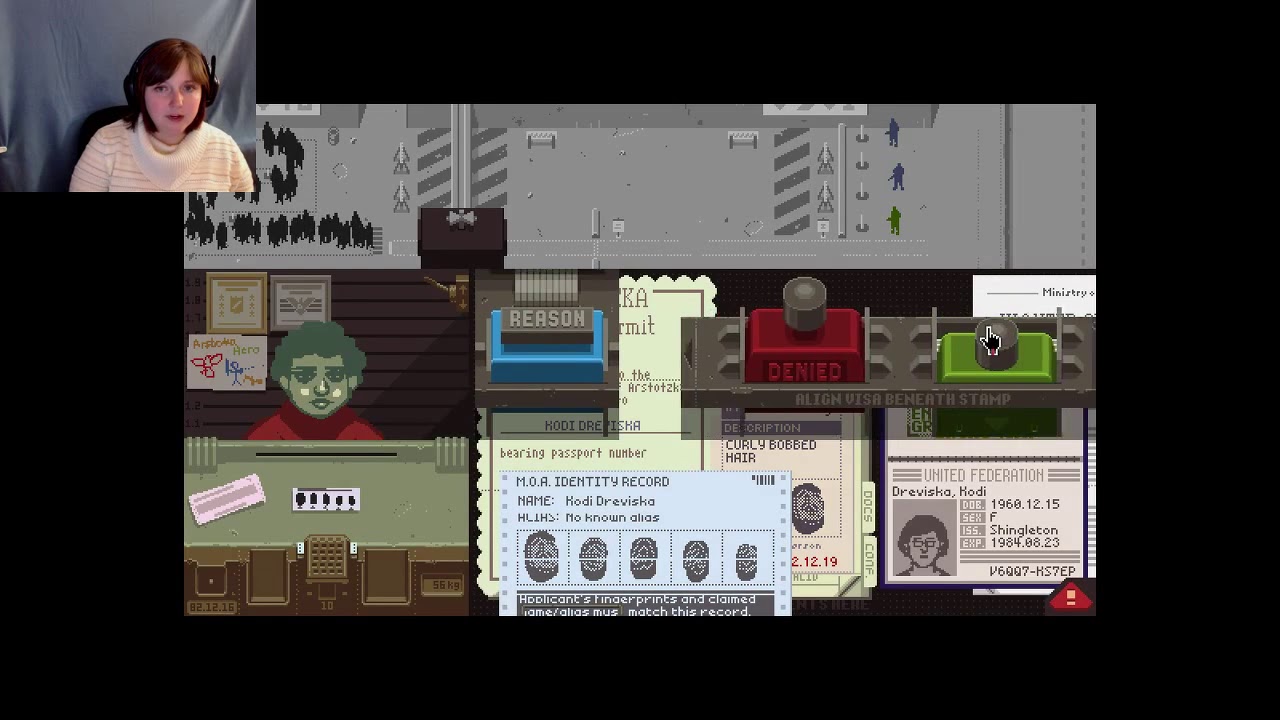In this detailed image, we see a Caucasian female streamer in the top left corner, identified by her brown hair parted in the middle, wearing a white turtleneck sweater with gold horizontal stripes, and a black headset. She is playing the game 'Papers, Please,' which involves working at an immigration checkpoint. The backdrop behind her is a blue-gray drape. The game's interface, occupying the main part of the image, features various sections including silhouettes of people lined up in front of a security checkpoint at the top, indicating they are waiting to be processed. The middle section showcases an immigration booth with documents such as a passport on the left, containing details like name and personal data, and stamps for approval or denial on the right. The bottom of the screen displays additional passport details, like a person's identity record, fingerprints, and a United Federation badge. The visual elements suggest the intense and potentially controversial nature of the game, as players must scrutinize documents and decide whether to grant or deny entry to individuals based on various criteria.